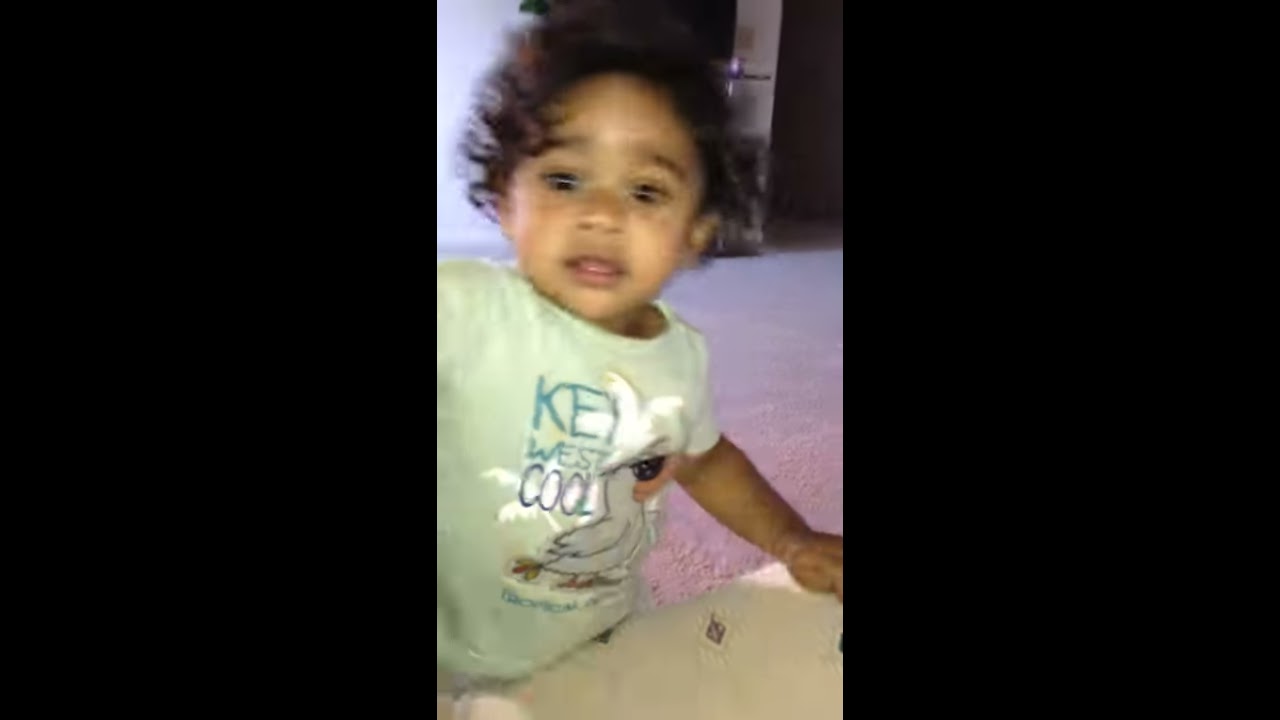This image captures a detailed yet slightly blurry photograph of a surprised toddler with short, curly brown hair and expressive brown eyes. They have a light green shirt on featuring the text "Key West Cool" alongside a colorful bird illustration that showcases yellow and red tail feathers, orange feet, and an orange beak with sunglasses. The child, appearing either to be standing or leaning with one hand on what seems to be a white or beige sofa, bench, or table, has an open-mouthed expression suggesting a blend of curiosity and astonishment. 

The backdrop includes a living room setting with pinkish-hued carpeting extending to a partially sunlit area with white and brown wall elements. The photo's blurred quality and the darkened bands along the sides enhance the central focus on the child, whose pleasant yet surprised look makes them the undeniable focal point of the image. One of the child's arms is notably positioned off-frame, adding to the intriguing composition of the scene.